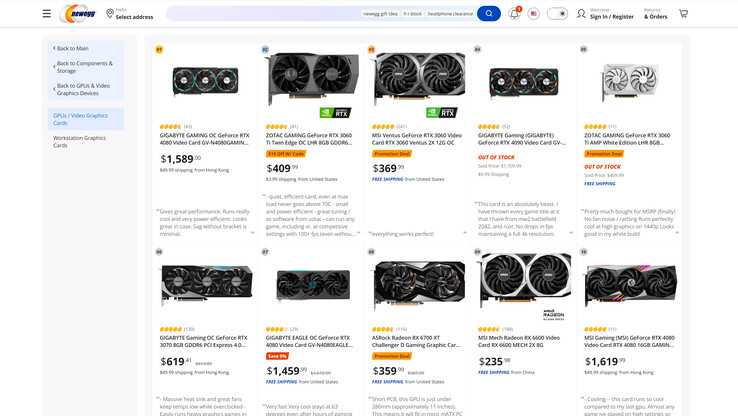Screenshot featuring an interface with a white background. At the top, there is a location symbol followed by the text "Hello, Select Address." Next to it is a blue circle containing a white magnifying glass, indicating a search feature. To the right of the search icon, there's a notification bell with a red badge displaying a number, possibly 9 or 1. Below this, there is a U.S. map icon beside the text "Sign In / Register" accompanied by an outline of a user profile picture. Further to the right, there are options labeled "Returns & Orders" and a shopping cart icon. Above the "Sign In / Register" text, there is the word "Welcome." 

The main section displays several product images, likely video cards, with detailed prices. The first product is priced at $1,589. The second product is listed at $409.99, followed by another priced at $369.99. Some items are marked as "Out of Stock". This layout suggests a user interface for an online shopping platform, presenting various options and product details, predominantly video cards.